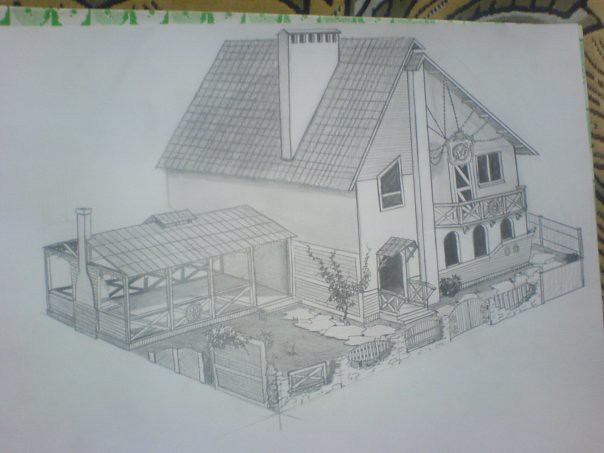A meticulously hand-drawn pencil sketch of a sizable house is presented on a large, unlined white sheet of paper. The paper rests on a green and white surface, which in turn appears to lie atop a yellow, white, and gray patterned base. The house itself boasts a number of intricate architectural features. It has a slanted roof with a distinct line running down the front above one of the windows, adding to the overall texture of the facade. Hanging from some chains is an elaborate object, adding a touch of whimsical charm. One side of the house showcases a balcony adorned with exquisite carvings, contributing to the grandeur of the residence. Below, there are detailed wooden carvings in front of the windows, enhancing the artistic value of the sketch. The doorway is highlighted by an awning that provides a quaint entry point, with wooden railings adjacent to it. To the side, a sunroom with a roof and screened doors adds a cozy extension to the house. In front of the house, there is a fence that provides a boundary, accompanied by thoughtfully sketched plants that bring the scene to life.